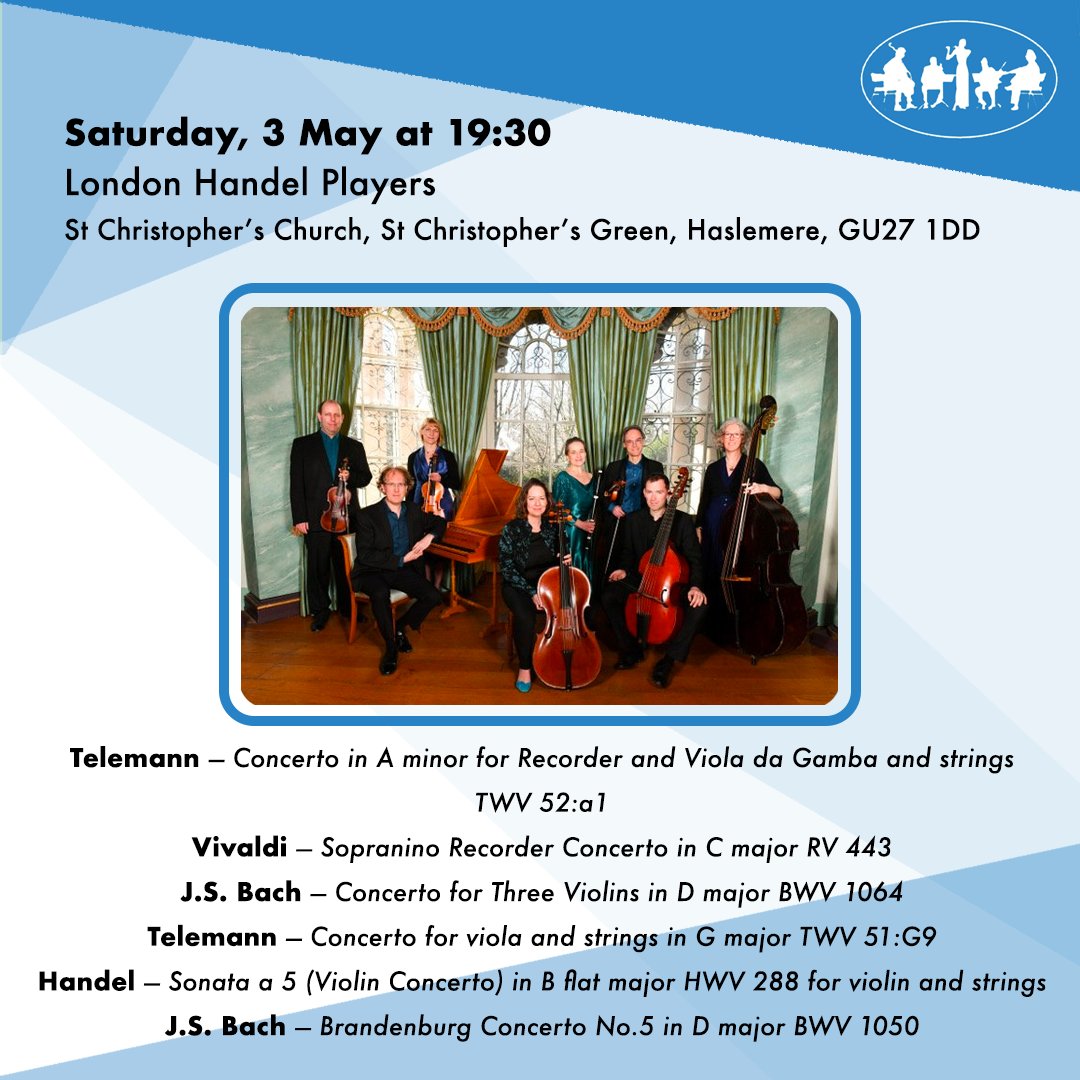The poster is a detailed, digital flyer featuring an advertisement for an orchestral performance by the London Handel Players. The background is a striking design composed of various shades of blue triangles, giving it an abstract, modern aesthetic. At the top left of the poster, in black text, it states the event date and time: "Saturday, 3 May at 19.30". Below this, it lists the performers and venue: "London Handel Players", "St. Christopher's Church, St. Christopher's Green, Haslemere, GU27 1DD".

The central portion of the poster showcases an image of the ensemble against the blue backdrop. In the foreground, several musicians are visible, including four violinists, three cello players, and an oboe player. On the very left, a man sits on a piano stool, in front of a wooden piano.

Below the image, the poster details the program for the evening, including pieces by renowned composers such as Telemann, Vivaldi, and Bach. Specific works listed include Telemann's Concerto in A Minor for Recorder and Strings, Vivaldi's Soprano Recorder Concerto in C Major, J.S. Bach's Concerto for 3 Violins in D Major, and Handel's Sonata at 5, among others. The detailed text provides a comprehensive overview of the event, ultimately enticing classical music enthusiasts to this performance.